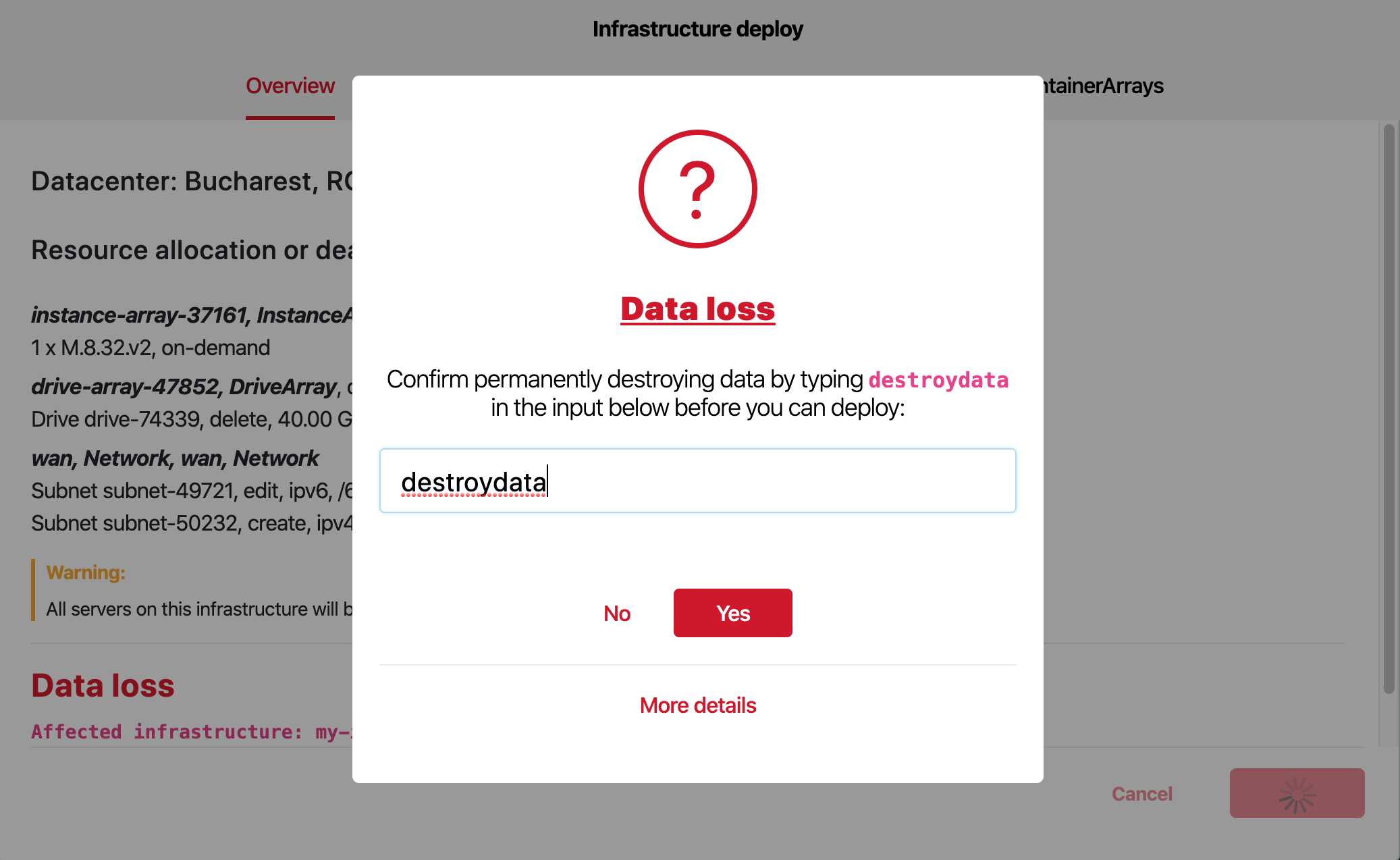The image appears to capture a webpage or app interface displaying a critical pop-up notification. At the center top of the screen, there is a red question mark encased within a white circular background bordered in red. Directly beneath this icon, the phrase "Data Loss" is prominently underlined in red. Following this header, the main body of the pop-up includes black text that reads: "Confirm permanently destroying data by typing." Below this instruction, the term "destroydata" is presented in neon pink, all lowercase letters. 

Further instructions specify that "destroydata" needs to be typed in an input box below, a prerequisite action before proceeding with deployment. This input box is outlined in blue, and within it, "destroydata" is already typed out in black text, with a cursor positioned immediately to the right. Underneath the typed text, several red dots are visible, suggesting that a spell check feature has been activated.

Towards the bottom of the pop-up, there are two buttons; the first button simply labeled "No," and the second button, labeled "Yes," features white text on a red background with rounded corners. These buttons are separated from the input area by a horizontal gray line. Finally, the phrase "More details" is located at the very bottom of the pop-up in red text.